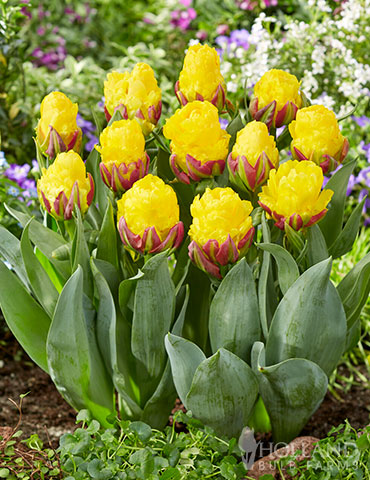This image showcases a vibrant and well-maintained patch of flowers, primarily featuring tall, chunky yellow blossoms that mimic the appearance of ice cream scoops nestled in red cups. Their eye-catching petals, lush and full, give an impression of being filled with butter. These striking flowers are surrounded by green leaves with a frosted tint and accompanied by feathery grasses in the foreground. The background reveals a sprinkling of smaller flowers in white, lavender, and magenta, lending a soft, colorful backdrop to the focal point. Despite not being in focus, this mix enhances the overall beauty and depth of the scene. The setting suggests a professional cultivation, perhaps indicated by the watermark of the Holland Bulb Company, and the arrangement includes elements reminiscent of tulip leaves, giving an impression of either an aloe variety or tulip hybrid. The rectangular composition captures an exquisite floral display, exuding freshness and exceptional care.